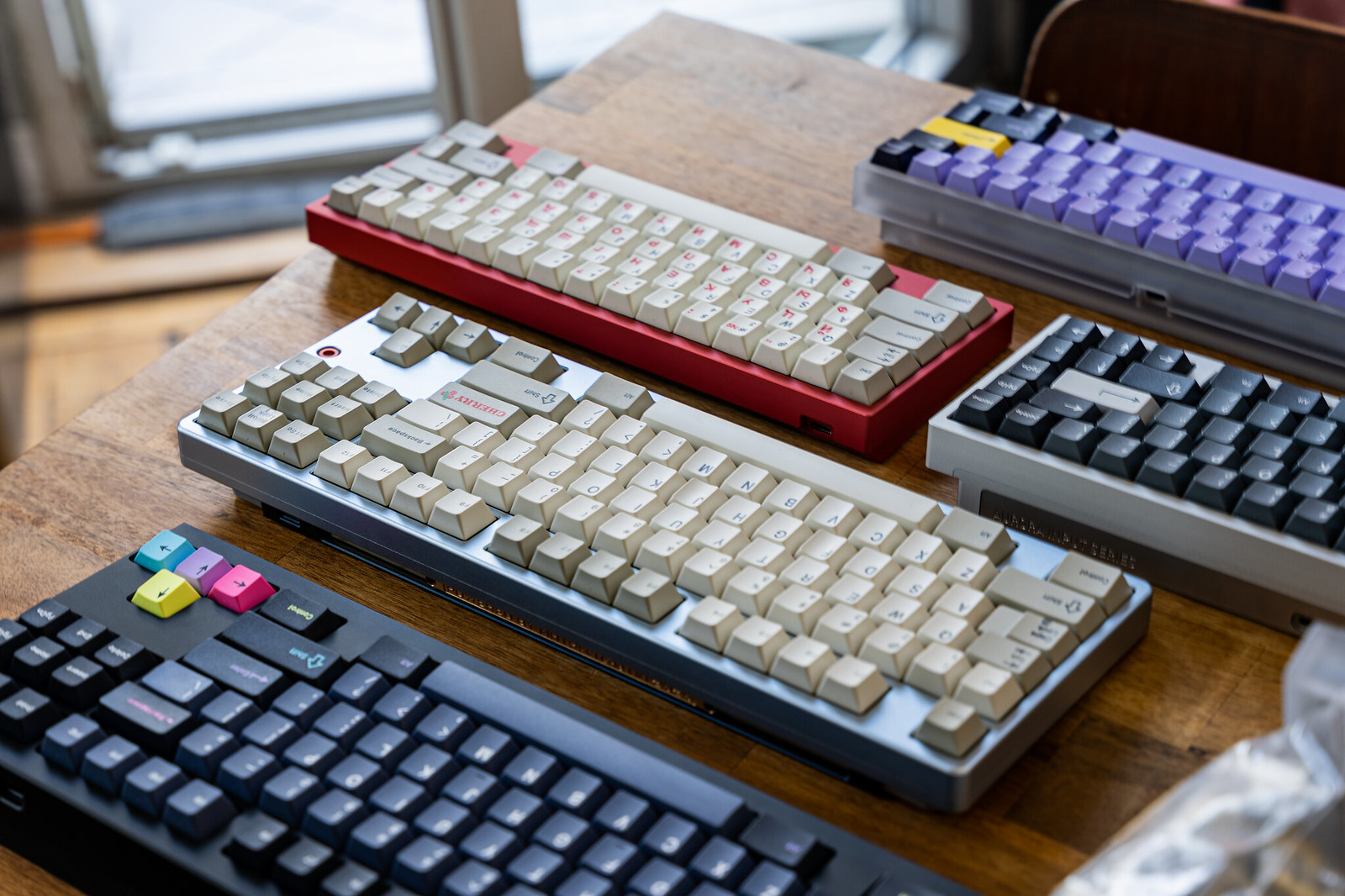This is a detailed photograph of five distinct computer keyboards arranged on a rough, older wooden desk, likely in a home setting with blurred windows visible in the background. The keyboards, which are mechanical with large, prominent keys, show signs of use and age, suggesting they are vintage models. 

Starting from the top:
1. A keyboard with blue keys and a gray base.
2. Below it, partially to the left, is a keyboard with white keys and a red base.
3. Directly to the right of that is another keyboard with black keys on a gray base.
4. Further down is a keyboard with white keys and a light bluish base.
5. At the bottom left, a striking keyboard with a black base and multicolored arrow keys in yellow, blue, purple, and pink stands out.

These keyboards are not connected to any computers or devices, and there is a plastic bag visible towards the bottom right of the desk. An old chair is positioned against the table, emphasizing the overall vintage atmosphere of the setting.